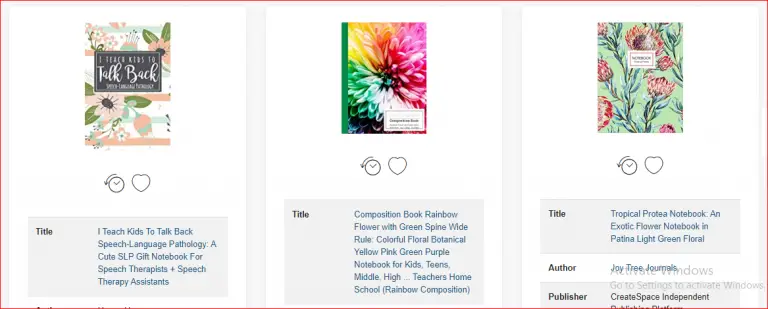The rectangular horizontal image features a thin red border surrounding it. The main background is light gray, with three distinct white vertical boxes evenly distributed across the image—one on the left, one in the center, and one on the right.

**Left Section:**
- **Top-left Image:** A colorful book cover featuring green, white, and red stripes. Pink roses adorn the top-right and bottom-left corners of the book cover.
- **Center Box:** A gray box containing text, accompanied by a heart emoticon and a small clock to the left.
- **Bottom Box:** A light gray box with the title of the book. The word "Titles" is on the left side, and the book title, outlined in blue, is on the right.

**Center Section:**
- **Top-center Image:** A vivid book cover resembling a colorful flower, showcasing hues of pink, orange, yellow, green, blue, and red. The spine of the book is dark green.
- **Bottom Box:** Below the book, similar emoticons as in the left section appear. A blue-outlined title of the book is displayed to the right of the word "Titles."

**Right Section:**
- **Top-right Image:** A green book cover decorated with intricate green vines and flowering elements.
- **Bottom Box:** Emoticons are featured beneath the book cover, and again the title of the book in blue is found to the right of the bold word "Titles." Additionally, this section includes the author name in blue and the publisher name in black.

The composition effectively segments the visual information, allowing clear differentiation between each book's cover design and associated details.